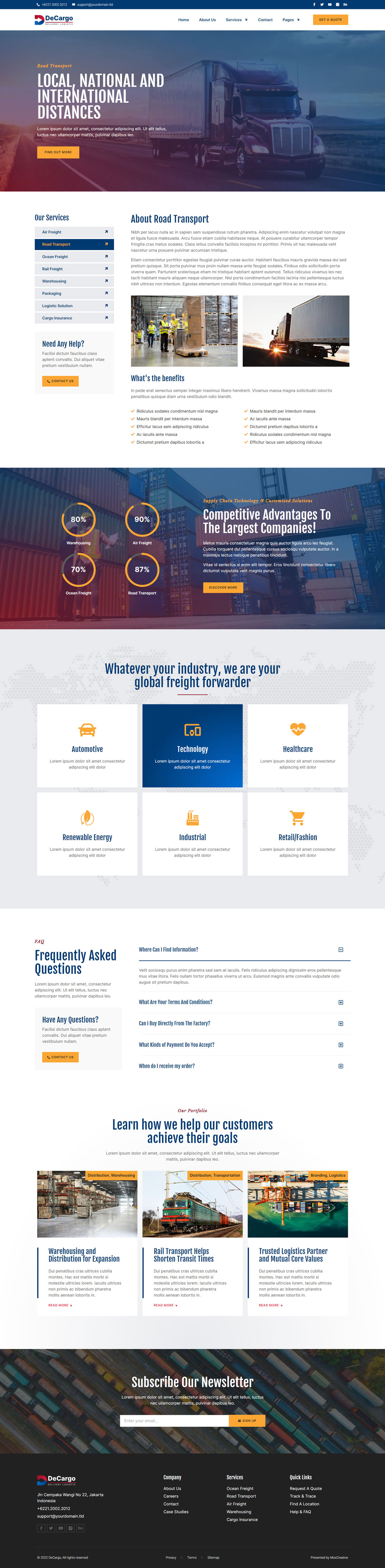This detailed caption provides a comprehensive description of the website's layout, visuals, and content elements:

---

The screenshot depicts a comprehensive truck driving information website. Dominated by a large and lengthy layout, the website features a photograph of an 18-wheeler truck, centrally positioned on a road, with blue and red tones. Overlaying this image is the text "Local, National and International Distances" in a bold white font.

Adjacent to the photograph, a noticeable yellow-golden triangle acts as an interactive element for users to click for additional details. Below this section, there is an extensive article about road transport, presented as a large block of text. Along the sides of the article, there are navigational options allowing users to select specific topics of interest.

The website includes thumbnail images: one depicting workers in yellow vests and black pants, and another showing a truck driver moving away with the sun setting on the horizon. This imagery accentuates the article "Competitive Advantages to the Largest Companies." Beside these visuals are partially completed circles displaying percentages of 80%, 90%, 87%, and 70%, although the text detailing their significance is too small to read.

Further down, the tagline "Whatever Your Industry, We Are Your Global Freight Forwarder" is presented alongside six clickable rectangles, arranged in a 3x2 grid. The bottom section of the webpage offers a list of frequently asked questions with corresponding answers, encouraging users to "Learn How We Help Our Customers Achieve Their Goals." Additional clickable images of trucks provide further opportunities to explore supporting articles.

---